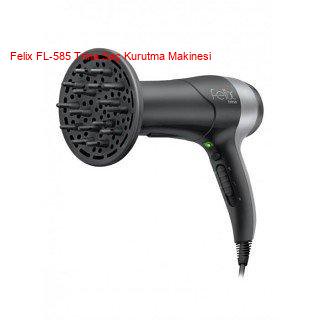This detailed image features a sleek black hairdryer with a silver stripe towards the back. It prominently includes a diffuser attachment on its nozzle, distinguished by several long prongs and both circular and rectangular perforations, designed for efficiently drying curly hair. The background is solid white, emphasizing the hairdryer's design. The hairdryer faces left, displaying its logo, "Felix," near the silver section at the back, along with some very small, unreadable text below it. A green button or light is visible on the handle, which slightly tapers where the cord, only barely visible, connects. Above the hairdryer, in red text partially obscured by the device itself, is the model name "Felix FL-585," followed by the words "Kurutma Makinesi," suggesting the description of its function in another language.